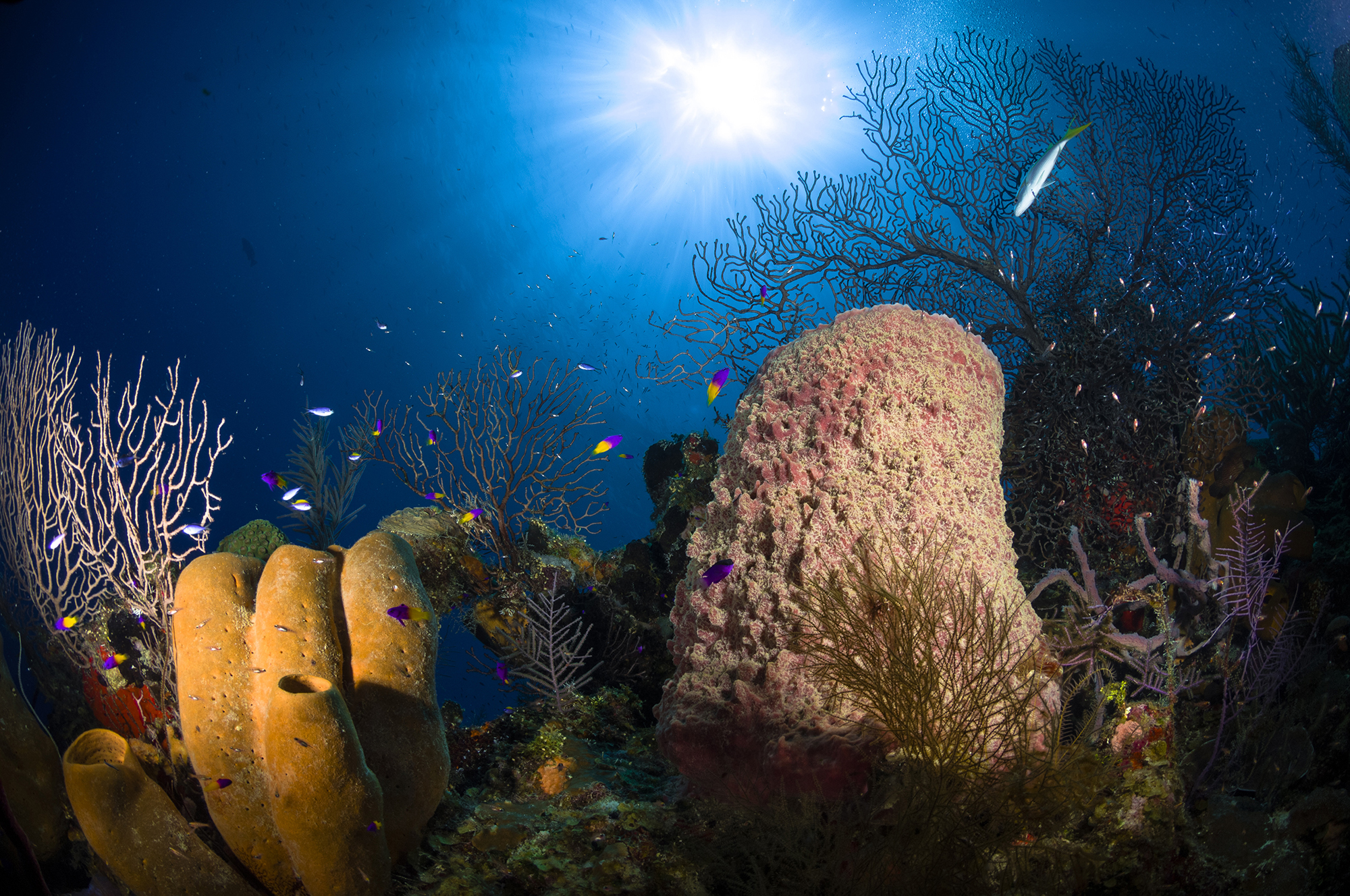This vivid underwater scene, captured from the perspective of a diver on the ocean floor, showcases the sun's rays piercing through the deep blue water, illuminating a colorful coral reef. The seabed is adorned with a diversity of coral structures: large yellow and pinkish-white corals dominate the scene, with tree-like coral formations branching off in various directions. In the lower left corner, yellow tube-shaped coral stands out, while pink, rocky-looking coral adds another layer of texture. The upper corners feature taller, darker coral with purplish hues. Tiny yellow and purple fish dart around the reef, accompanied by two distinct blue and yellow fish, as well as a white and yellow fish, all contributing to the lively underwater tableau. The background, filled with vibrant blue water, enhances the scene's depth and the sun's radiant glow.